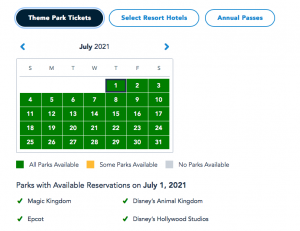In the image displayed on a computer screen, there is a detailed calendar interface for July 2021. At the top of the screen, three oval buttons are visible, with the left one highlighted in black, indicating it has been selected. This button is labeled "Theme Park Tickets."

Below the top part, a monthly calendar for July 2021 is presented. The entire grid of dates from July 1st to July 31st is colored green with white numbers, signifying park availability. Underneath the calendar, there is a legend explaining the color coding: green squares indicate that all parks are available, yellow squares signify that some parks are available, and gray squares show that no parks are available.

Further down, in black text, the caption reads "Parks with available reservations on July 1st, 2021." Below this text, there is a list of the theme parks with checkmarks next to each one, including Magic Kingdom, Epcot, Disney's Animal Kingdom, and Disney's Hollywood Studios, confirming their availability. The image suggests that someone is in the process of booking tickets for one of the Disney theme parks, with all dates in July being open for reservation across all parks.